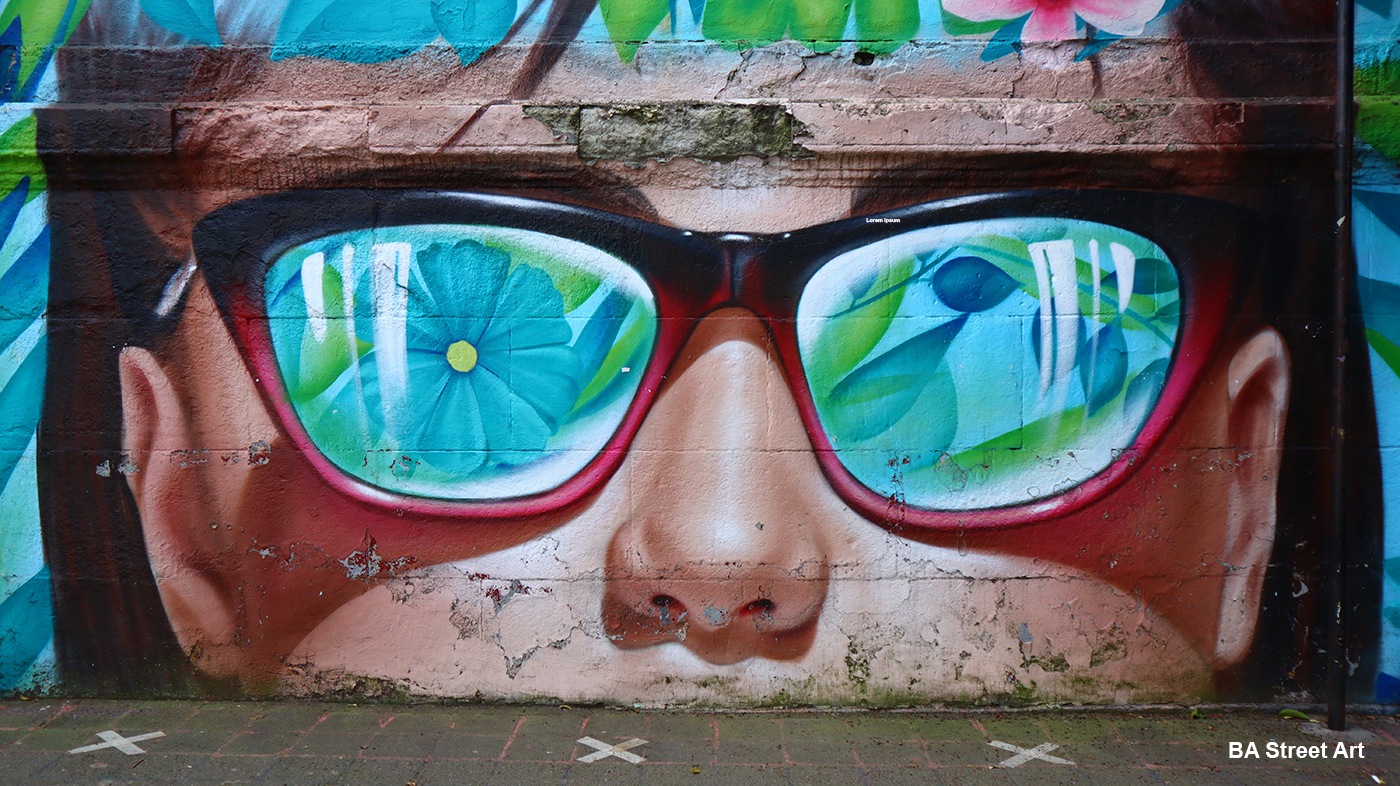This artwork is a vibrant street mural occupying an entire brick wall. The mural depicts a close-up of a young man's face, from the nose to the forehead, adorned with colorful glasses. These glasses, black on top and pinkish-red on the bottom, vividly reflect blue flowers with petals and stems. The skin is portrayed in a flesh tone, and the young man’s face appears dirty. Surrounding the head are artistic renderings of foliage and flowers, covering parts of the forehead. The mural is set against the textured background of the brick wall, enhancing the details, such as the changing lines where the bricks are located. In the bottom right corner of the mural, the text "B.A. Street Art" is prominently displayed. The mural appears to be viewed through a wooden box with three white X's at the bottom.